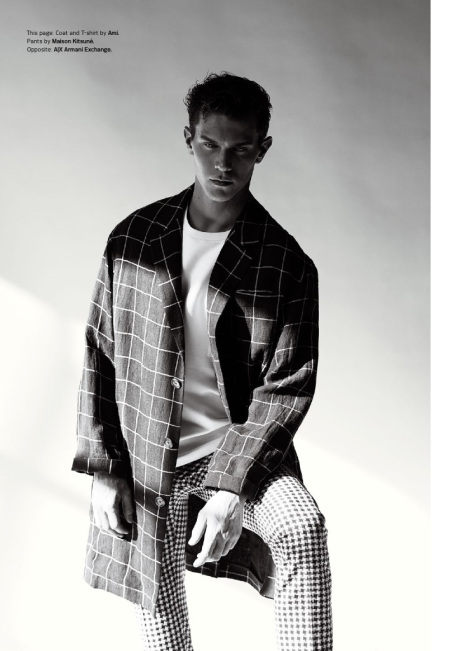The image is a black and white photograph featuring a young Caucasian male model with a well-built physique. He is depicted wearing an elongated, checkered overcoat, coupled with matching checkered pants and a white undershirt. His short black hair is neatly styled, and his clean-shaven face bears a stern, serious expression as he looks off into the distance. The lighting, primarily coming from the left side, illuminates the lower part of the image, adding contrast to the scene. There is blurred black text in the upper left corner, making it difficult to read against the white background.